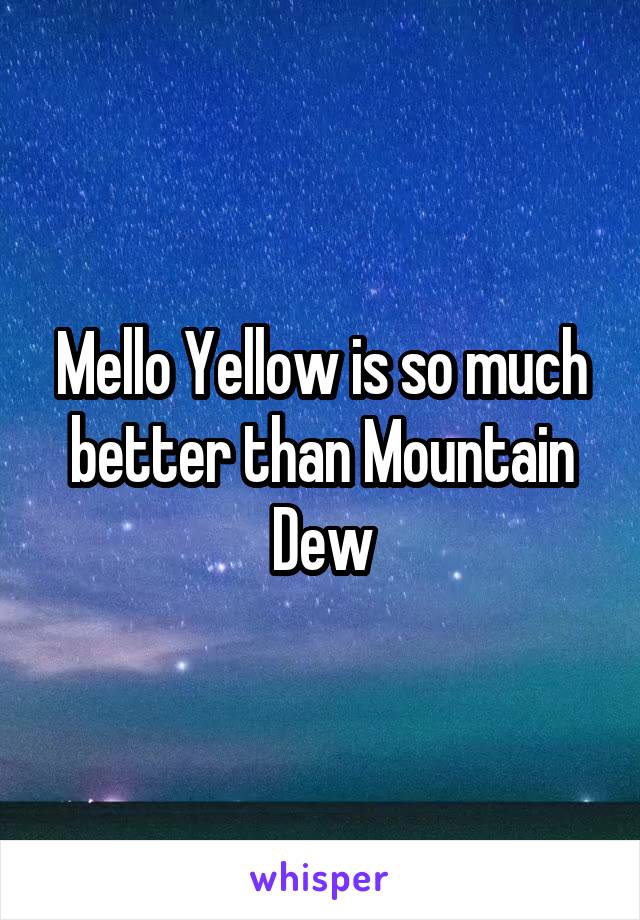The image is a color photograph of a twilight sky transitioning from a bright aqua blue near the horizon to a deeper blue with thousands of stars scattered across the top. Below the sky, you can see the faint outline of a large body of water, possibly the ocean, with some indistinct lights near the horizon that could be ships or distant buildings. Just above the horizon, the last rays of the setting sun are visible, indicating the very end of twilight. In the middle of the image, bold white text with black borders declares, "Mellow Yellow is so much better than Mountain Dew." Overlaid near the bottom is the word "Whisper" in purple text, resembling a logo rather than an audible whisper.